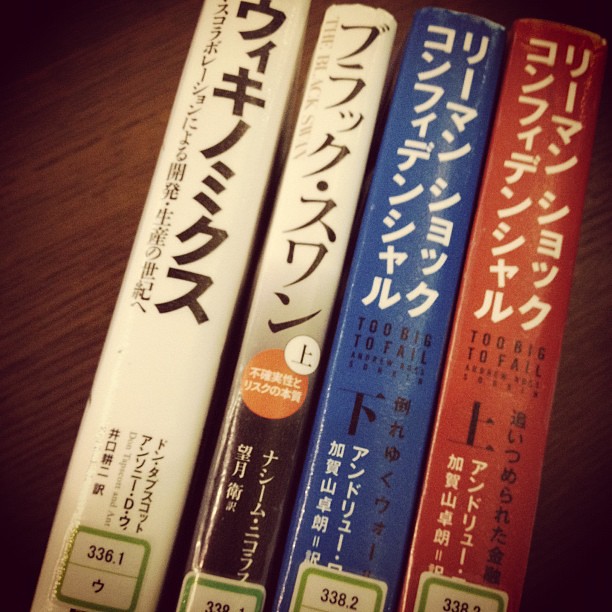The image captures four vertically positioned books arranged on a dark brown walnut table, seen from a top-down angle. The titles are all in Japanese, with two books featuring English subtitles. The books lie tilted slightly to the right. On the far left is a white-spined book with black lettering, featuring a green label reading "336.1" on the bottom. Next to it is a book with a white upper spine transitioning to black on the bottom, interrupted by an orange circle and a green label, though the Dewey Decimal number is partially obscured. Following this is a blue book with "Too Big to Fail" in English and a green library sticker marked "338.2". The final book is red with the same English title "Too Big to Fail," accompanied by Japanese text and a partially visible green sticker, likely ending in "338". The books exhibit minor wear but are in generally good condition, suggesting they are library books, as evidenced by the Dewey Decimal labels and other library markings.